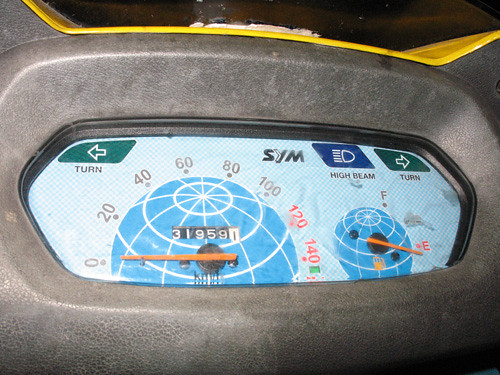The image captures a close-up view of a compact digital display, most likely from a motorcycle dashboard. Dominating the screen is a blue-toned globe-like design, centered around a prominent odometer reading of "31,959" displayed in white letters against black squares. Surrounding the odometer are speed indicators marked in an ascending order of 20, 40, 60, 80, and 100 in black numerals, with the 120 and 140 highlighted in red. An orange needle points out the current speed, adding clarity to the gauge's functionality.

Adjacent to the main speedometer, there’s a smaller circular gauge with another orange needle pointing between the letters 'F' (Full) at the top and 'E' (Empty) at the bottom, signifying the fuel level indicator. In the top left corner, a directional arrow pointing left is paired with the word "turn," indicating the left turn signal, while on the opposite side, a similar right-facing arrow denotes the right turn signal. Both turn signal indicators are green. Additionally, a blue high beam icon is situated nearby, signifying the activation of the high beam headlights.

This image provides an intricate and detailed look at a specialized vehicular dashboard, likely from a motorcycle, characterized by its intuitive layout and color-coded indicators for efficient navigation and operation.